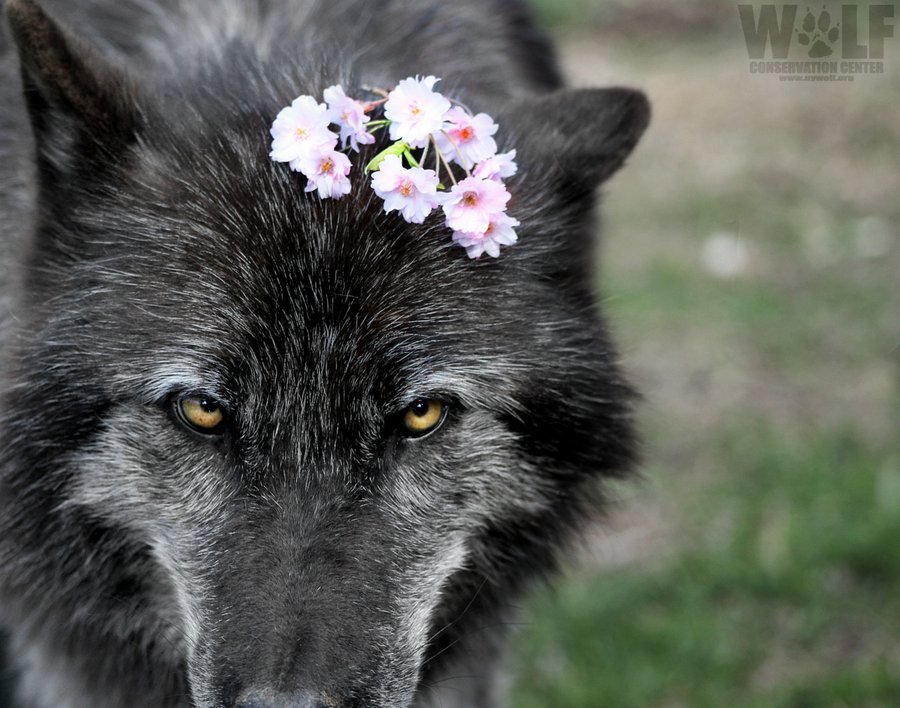The image is a large, square close-up of a fierce, predominantly black and white wolf's face, occupying the left side of the picture. The wolf's intense, gold-colored eyes with black centers are sharply in focus, looking up while the head is angled slightly downward. The top of the wolf's head is adorned with small white and pink flowers. The rest of the wolf's body is out of focus, blending into the background. The entire right side of the image is a blurry mix of green and brown grass. In the upper right corner, the word "WOLF" is prominently displayed in large, dark letters, with a paw print substituting for the letter "O." Beneath this, "Conservation Center" is written in smaller print, although part of the text is unclear.